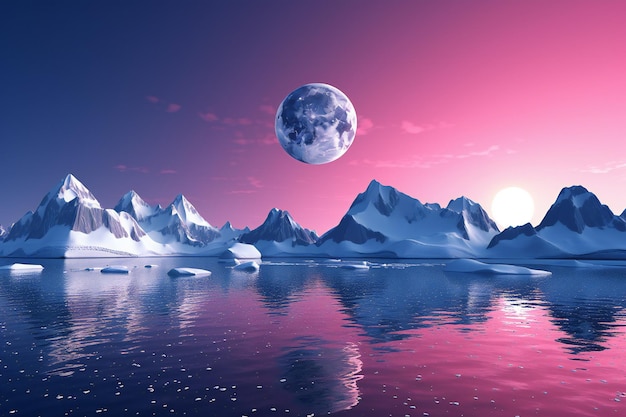This is a detailed digital artwork, portraying a surreal arctic landscape. The image is square with no borders or distinct background, focusing entirely on the artist's vivid interpretation. Dominating the top center is an abnormally large moon, surrounded by a sky that transitions from a dark blue, almost black hue on the left to a light purple and pinkish-orange on the right. Below the sky, a grand mountain range spans vertically across the middle, its peaks blanketed in grayish snow. Nestled between some mountains is a smaller, yellow sun peeking out, casting reflections in the calm waters below. The tranquil water is dotted with floating chunks of ice and mirrors the contrasting colors of the skies above, as well as the large moon. A thin layer of clouds lingers behind the moon, adding to the ethereal atmosphere of the scene.